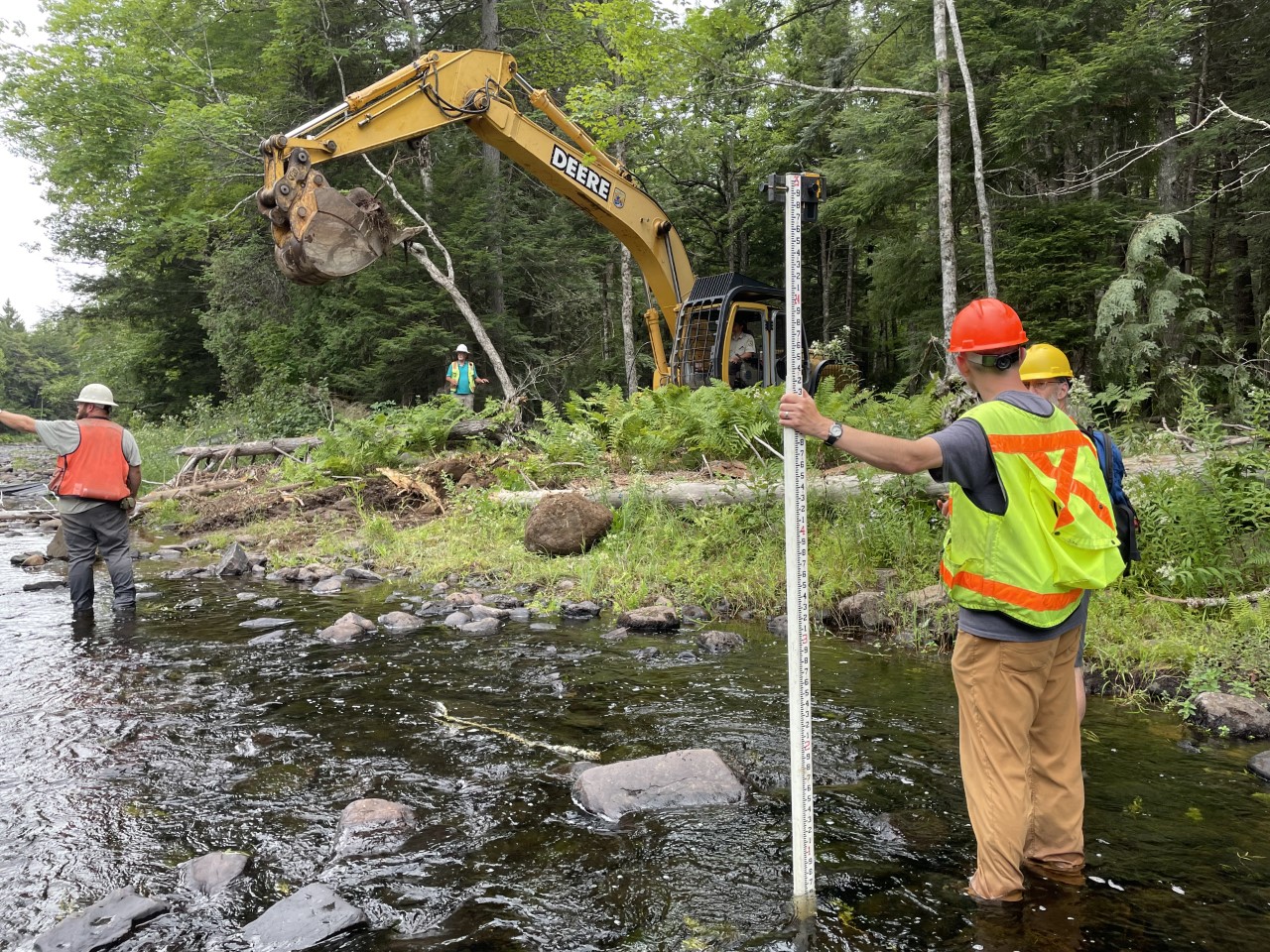In this color photograph of an outdoor maintenance or construction scene, various workers are engaged in what appears to be a cleanup or surveying operation by a shallow creek edged with lush, high grass, ferns, and fallen, decaying trees. The background is dominated by a line of indistinct trees. 

Towards the middle and left side of the image, three men stand in the creek. One of these men, wearing an orange construction helmet, khaki pants, a blue-gray shirt, and a yellow vest with an orange stripe, holds a tall measuring stick like a surveyor and converses with a nearby man, only partially visible, who dons a yellow helmet. Another man, further upstream and facing away, points towards the left edge of the photo. This man sports a white helmet, an orange vest over a gray shirt, and dark gray pants.

In the grassy area towards the top center, a large John Deere backhoe stands with its scoop raised, presumably filled with rocks and dirt. Below the arm of this yellow machine, yet another worker stands wearing a white helmet, a yellow vest over a turquoise shirt, and tan pants, appearing to be spotting or guiding the backhoe operator, who is not clearly visible. 

On the bottom right, two men are in conversation. One, wearing a red helmet, a light blue shirt, and a yellow-orange vest, seems to be discussing the work at hand with a man in a yellow helmet who is mostly obscured from view. 

The area also features numerous scattered rocks in the shallow creek, contributing to the slightly murky water, and is surrounded by abundant greenery and fallen trees, underscoring the ongoing efforts of the crew to manage the natural and structural elements of the landscape.